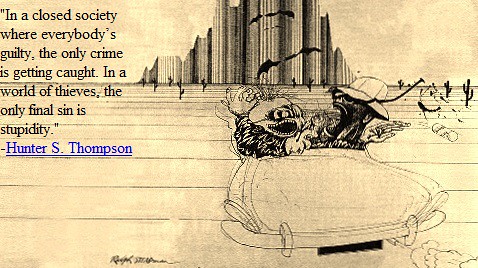In this small, horizontal, rectangular illustration by Hunter S. Thompson, set against a pale yellow, aged paper-like background with vertical stripes, two or three cartoon characters are seen driving a convertible. The car is rendered with just a visible outline, and the characters exhibit exaggerated, scribbly, and vibrant expressions typical of "Fear and Loathing in Las Vegas." They drive through an abstract desert landscape featuring cactuses, bats, and possibly splotches of paint in midair, with tall, geometric buildings or mountains in the background. On the upper left corner, a black typed-out quote reads, "In a closed society where everybody is guilty, the only crime is getting caught. In a world of thieves, the only final sin is stupidity." Beneath this quote, in blue text, is the attribution to Hunter S. Thompson.